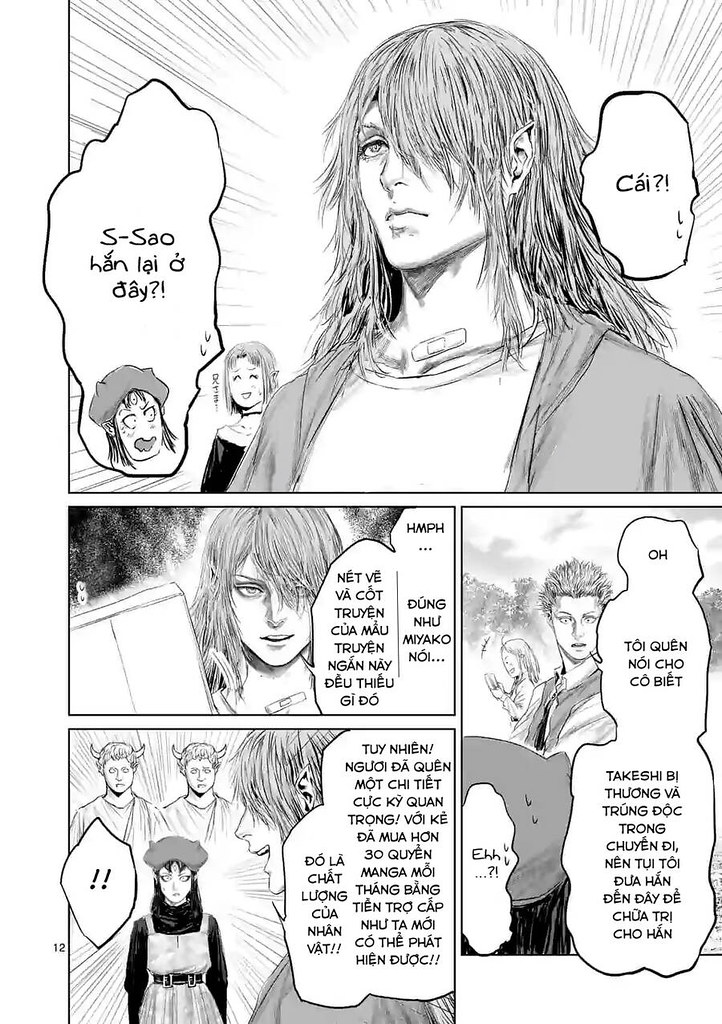The image features a detailed black-and-white comic book or manga page with multiple panels. The top panel, which occupies a significant portion, depicts a man with long hair obscuring his face, pointy ears, and a bandage on his neck. He is surrounded by two speech bubbles: the left one reads "Es sao han lai oe?" while the right one says "Kai?" or "CAI?" with a question mark and exclamation mark. Behind this man, partially visible over his shoulder, is another person. The middle section contains three panels. The leftmost panel shows a person with two thought bubbles, one of which has the text "Hm... Dong nui mia ko noi?" There are additional texts like "Net ve va kat? Tru yen kua muau? Tru yen ngnan ne diu thiu gi dou?" In the same middle section, two men with devil horns stand behind a confused-looking woman wearing a dark shirt and dress, her look emphasized by double exclamation marks beside her head. A speech bubble from the man in the first panel extends into this scene. The bottom section features a panel with a man sporting spiky hair and a mischievous child behind him, accompanied by unreadable speech bubbles. The overall composition depicts various interactions and expressions, suggesting a complex narrative with supernatural elements.